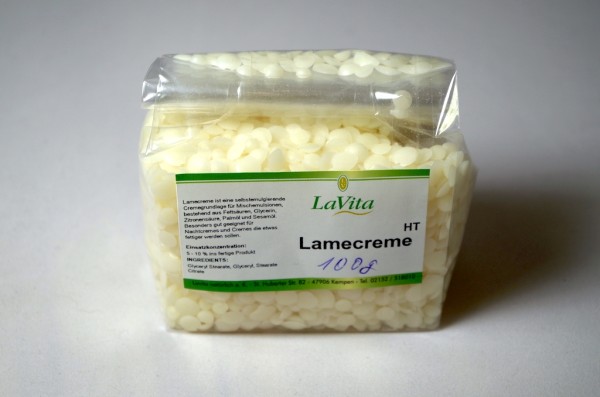This image shows a photo of a clear plastic cellophane bag containing numerous small, cream-colored pellets. The bag is rolled down at the top and has a distinct label in its center. The label is white with green borders on both the top and bottom edges. Prominently displayed in green text on the label is the brand name "LaVita," accompanied by a yellow oval symbol above the letter "V" and a wavy swoosh mark below it. Directly beneath "LaVita" in black font is the text "Lame Creme," with "HT" written above the letter "E." Handwritten in ballpoint pen, the label also indicates "100G." Although there are additional details on the left side of the label, such as ingredients, they are too small to be legible in the image. The scene is set against a white table or countertop with subtle gray shadows providing contrast.